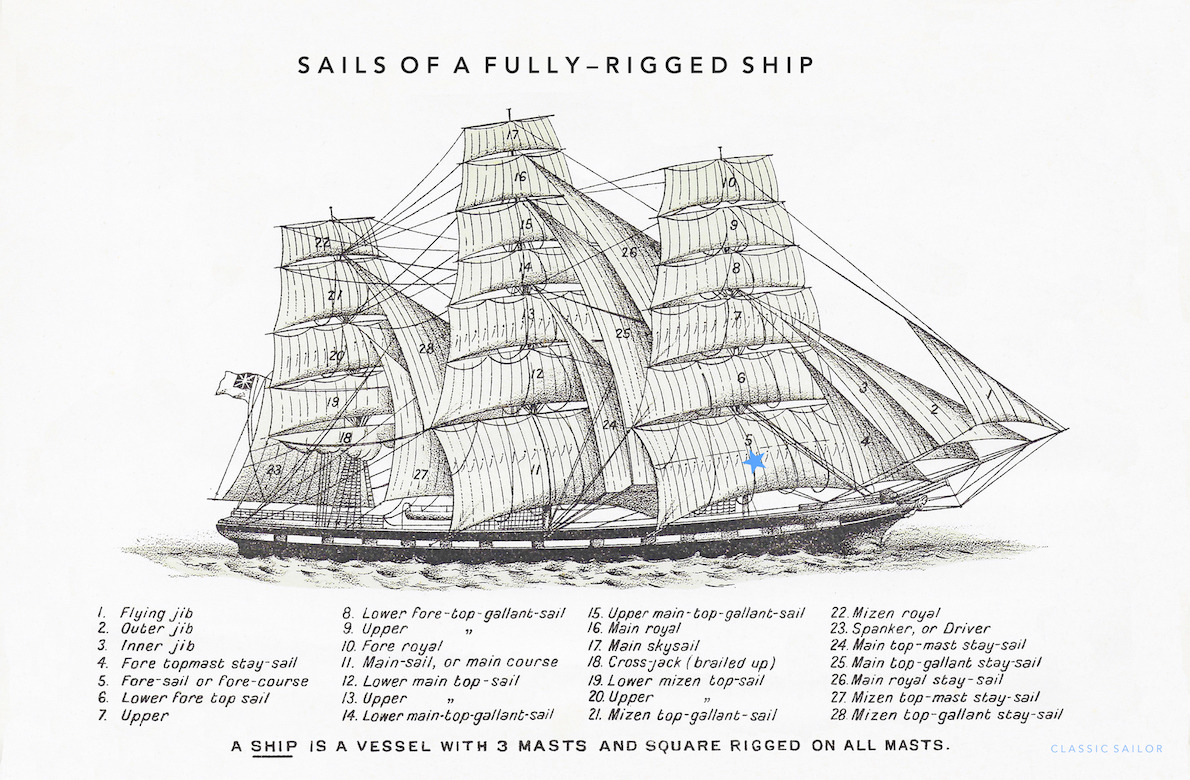The image is a highly detailed, black and white pencil sketch titled "Sails of a Fully Rigged Ship." It features a large, three-masted sailing vessel, square-rigged on all its masts. Each sail is individually numbered and labeled, with the numbering system described in detail at the bottom of the infographic. The ship, floating serenely on the sea, includes a flag, multiple decks, and an array of sails sequentially identified as follows: One, flying jib; Two, outer jib; Three, inner jib; Four, fore topmast staysail; Five, foresail or fore course; Six, lower fore topsail; Seven, upper fore topsail; Eight, lower fore topgallant sail; Nine, upper fore topgallant sail; Ten, fore royal; Eleven, mainsail or main course; Twelve, lower main topsail; Thirteen, upper main topsail; Fourteen, lower main topgallant sail, among others. A notable feature includes a blue star marking on sail number five. At the bottom of the image, it notes that "a ship is a vessel with three masts and square-rigged on all masts." Additionally, a watermark in the bottom right corner reads "Classic Sailor."